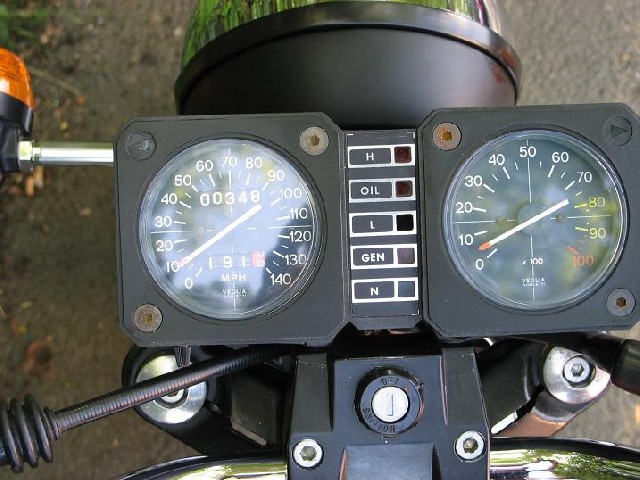The photograph is an overhead view of a motorcycle's dashboard and handlebars, set against a backdrop of asphalt interspersed with dried leaves and patches of grass on the left side. Prominently featured are two circular dials mounted on a square housing with visible bolts.

On the left, we have a speedometer with a white needle pointing below the 10 mph mark. The dial itself is graduated in increments of 10 from 0 to 140 mph. Beneath this are two odometer readouts – the top showing 00348 miles and the bottom displaying 191 miles, with a small red indicator for tenths of a mile.

To the right of the speedometer is another circular gauge, scaling from 0 to 100 with increments of 10, with the highest value, 100, in red. The gauge has a white needle tipped in red, though its exact function remains unspecified – possibly RPM.

Between the two dials, there is a narrow panel with several indicators including "H," "Oil," "L," "Gen," and "N." Below this panel is the ignition switch, which lacks a key.

At the top portion of the image, partially cropped off, is a headlight with a glass lens, and coming off to the left on a short chrome stem is a signal or directional light with an orange, cone-shaped lens seated in a black or brown Bakelite base.

Visible at the bottom of the image are the tops of the motorcycle’s fork tubes, each secured with a bolt, along with a glimpse of a possible lever for gear shifting and some chrome details likely belonging to the gas tank.